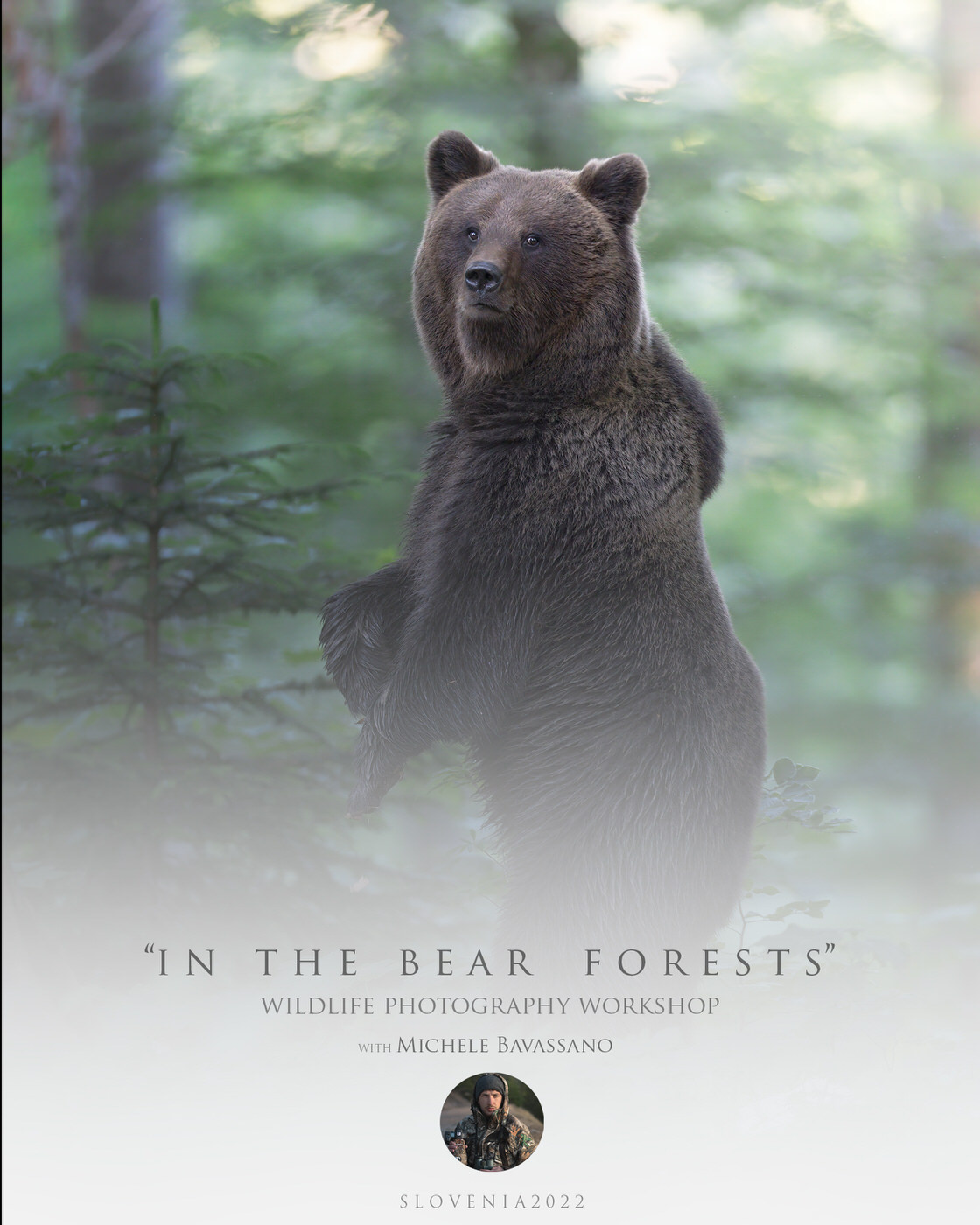This nature-themed advertisement features a striking image of a dark brown grizzly bear standing upright in a forest. The bear is sharply focused and looks directly at the viewer, appearing almost lifelike against a slightly faded and foggy forest backdrop, rich with greenery and various trees. Despite being taken during the day, the photo is not very luminous, contributing to its mystic atmosphere. The lower portion of the image features a text overlay in a white gradient, which reads: "In the Bear Forest, Wildlife Photography Workshop with Michel Bafassano, Slovenia 2022." Additionally, there is a round inset photograph at the bottom displaying a man in camouflage clothing, likely the photographer Michel Bafassano. This detailed and evocative poster captures the essence of wilderness and adventure, aimed at promoting a specialized photography workshop.